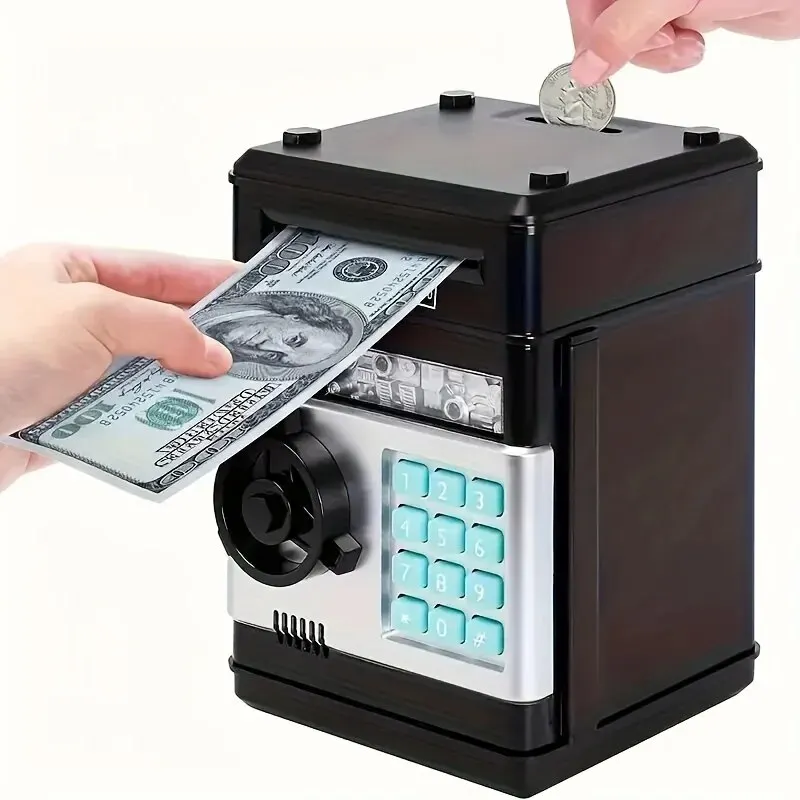This image depicts a modern yet antique-styled personal banking safe, designed for converting coins into cash notes. The device is centrally positioned, approximately six to eight inches tall, and rectangular in shape with a dark brown exterior. It features a teal and white numeric keypad on the front, alongside a black, round, spin-to-open handle, suggesting a blend of contemporary and traditional design elements. This safe also integrates a visible mechanism behind glass or plexiglass, enhancing its sophisticated appearance.

In the image, two hands are in action: one, appearing to have natural pink nail polish, is dropping a U.S. quarter into a coin slot at the top; the other, which is manicured, is inserting a $100 bill into a slot on the left side of the device. The detailed mechanics and security features such as the keypad and handle indicate a secure, functional device, likely intended for saving and converting spare change into more substantial denominations. This combination of elements and the carefully manicured hands suggest that the image may have been styled for sale or advertisement purposes, highlighting both the practicality and aesthetic appeal of the safe.